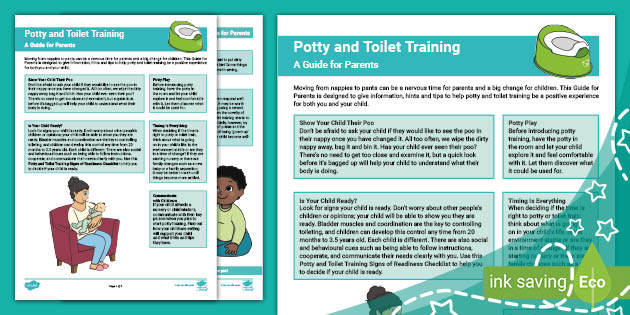The image depicts a detailed, single-page pamphlet focused on potty and toilet training, primarily colored in teal and turquoise hues. The pamphlet features a digital art style and is framed by a turquoise border, indicative of a digital format that may be viewed or turned like pages. The title "Potty and Toilet Training" is prominently displayed at the top, both in a teal banner on the left-hand side and in a similar section on the right-hand side, which also adds the subtitle "A Guide for Parents" alongside an illustration of a small green toilet.

Within the pamphlet, the left section reveals partial views of two overlapping pages. The visible portions include various rectangular and square boxes filled with text too small to decipher, likely providing practical instructions and advice on potty training. Among these elements, there is a noticeable illustration of a mother sitting in a red armchair, attentively holding a newborn baby, while another baby with dark hair and dark skin is visible, sitting up on the less exposed page.

On the right-hand side, additional rectangular and square text boxes offer more information, echoing the left-hand layout. Near the bottom right, set against a starry graphic, a green banner contains the words "ink saving eco," accompanied by an image of a leaf, emphasizing the pamphlet's environmentally friendly design. The coherent layout and the consistent teal theme underscore the pamphlet's purpose as a comprehensive, eco-conscious guide for parents on potty and toilet training their children.